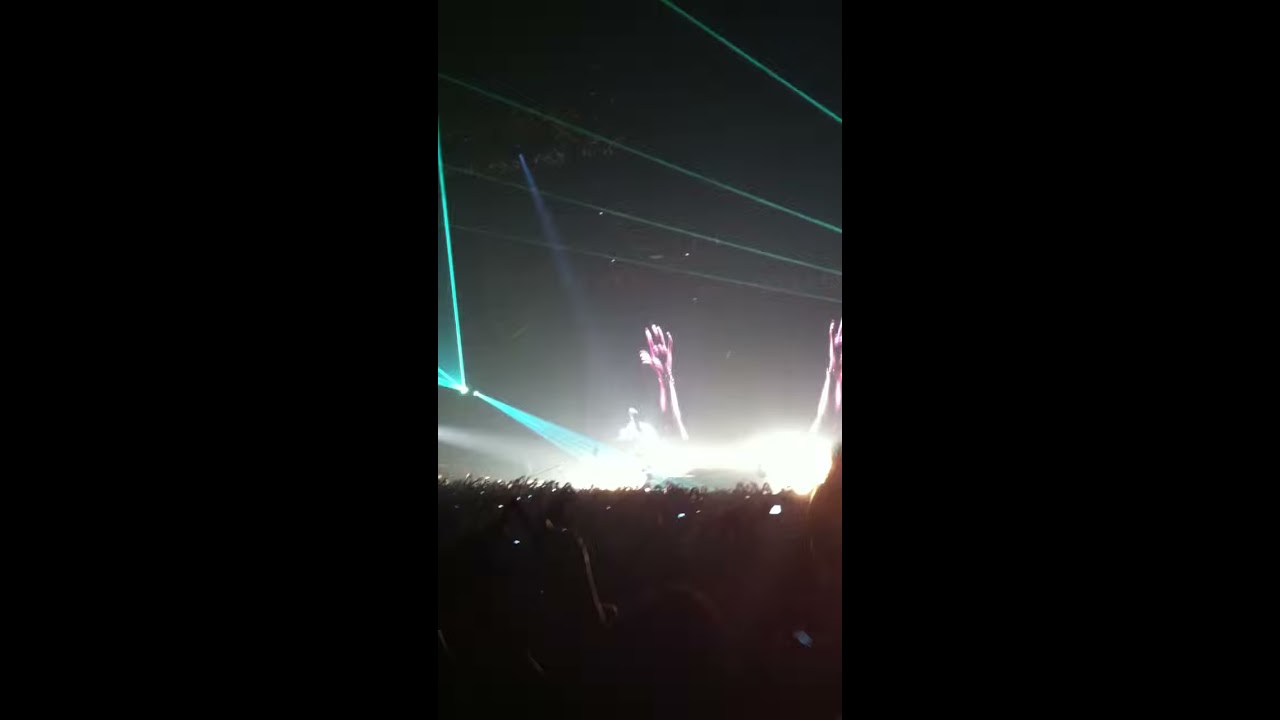The image captures an electrifying concert scene inside a vast, darkened stadium. The bottom half of the frame is dominated by an indistinct crowd, their presence signaled by the glow of countless cell phone screens raised to record the event. The stage, awash in powerful white light, is partially obscured, but a large screen behind it displays a silhouette of someone with arms outstretched. The dark ceiling of the venue, hidden in shadows, is intermittently pierced by vibrant green laser lights. Among these, a solitary white spotlight shines in the top left corner. With black support beams barely visible, the ceiling appears as a void. The ethereal glow of holographic-like red and pink hands or arms seem to float, reaching skyward, adding to the surreal atmosphere created by the intricate light show and overwhelming sense of scale and unity among the audience.